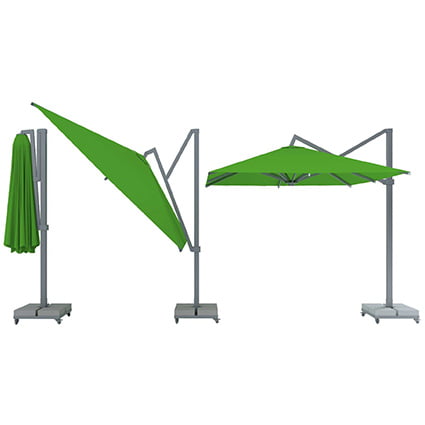This detailed color illustration in landscape orientation showcases a transportable awning, depicted in three stages of deployment. The sequence, from left to right, shows the awning folded, partially opened, and fully extended. The awning canopy is bright green, mounted on a vertical dark gray post featuring an arc at the top. The post is anchored on a wheeled, gray square platform, emphasizing its mobility. The leftmost image shows the awning folded compactly against the post. The middle image displays it halfway extended, and the rightmost image illustrates the awning fully opened to the left of the vertical post. The illustration floats on a white background, with no additional elements, likely aiming to highlight and perhaps market the awning’s functionality and design.